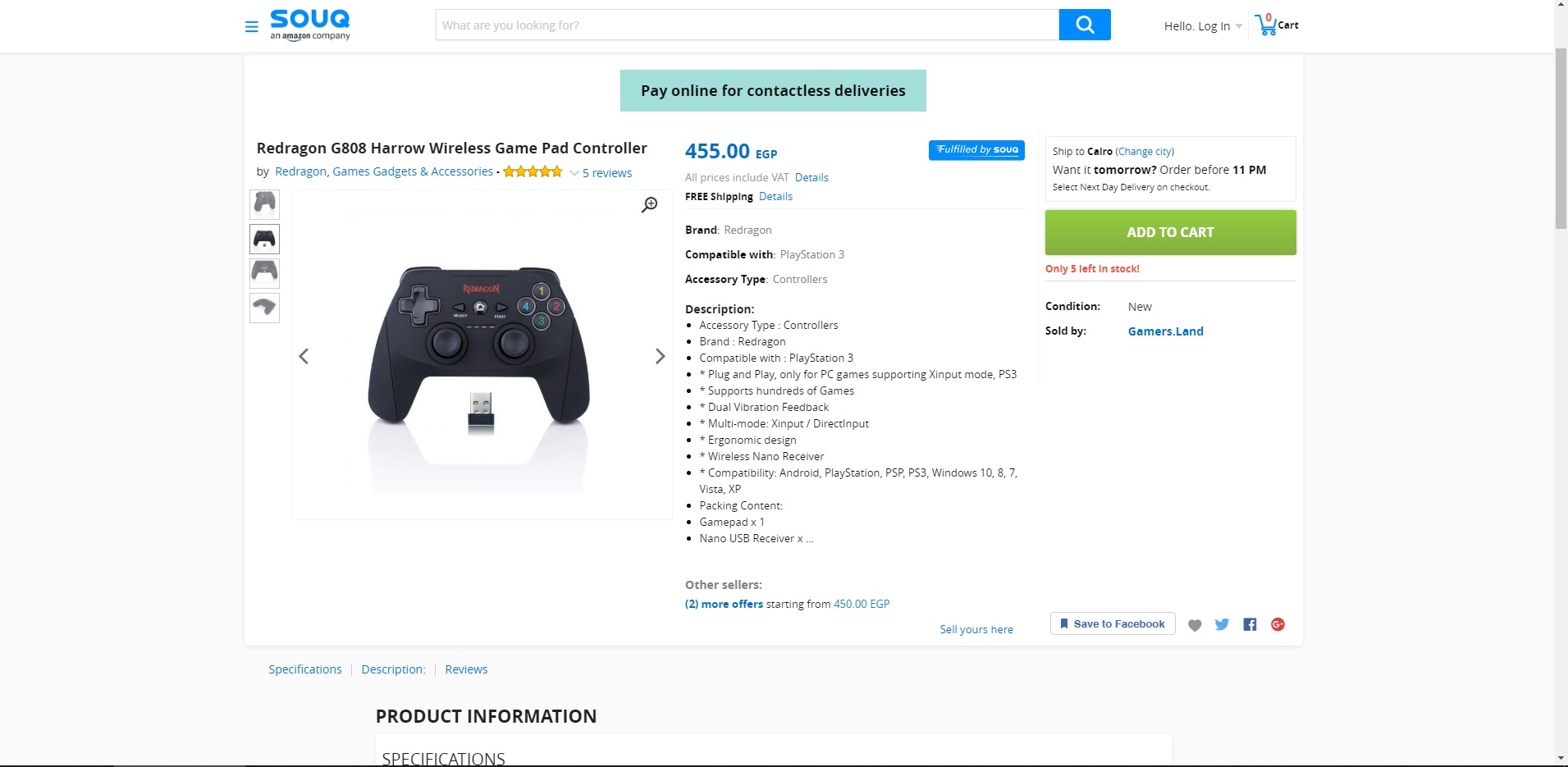This screenshot captures the homepage of Souq, an Amazon-owned website specializing in electronics and other devices. The page features a predominantly white background with text in black and blue colors. 

In the top left corner, the website's logo, "Souq" (spelled S-O-U-Q), is displayed in blue text. Beneath this logo, a tagline indicates its affiliation with Amazon. Centrally positioned at the top of the page, there is a search bar with the prompt "What are you looking for?" Inside the search bar, users can enter their search queries, and there is a blue search icon (a white magnifying glass) at the far right, which initiates the search.

The top right section of the page provides options for users to either log in to their accounts or view their shopping carts. The main focus of the page lies in the center, displaying a product listing for the "Redragon G808 HERO Wireless Gamepad Controller." The product name is highlighted in black text at the top left of this section. Below the product name, there is an image of the game controller itself—a black wireless controller featuring various multicolored buttons.

To the right of the controller image, a vertical column provides detailed information about the product. At the top, the price is listed in blue text: $455 EGP. This column includes various details such as the brand, compatibility, accessory type, and a thorough description of the game controller.

On the far right side of the page, another vertical column presents different purchasing and shipping options. A prominent green button with white text, labeled "Add to Cart," allows users to add the controller to their shopping cart for future purchase. This button is centrally placed in the right column.

The rest of the page includes additional links and information, such as social media icons and hyperlinks to other products available on the website.